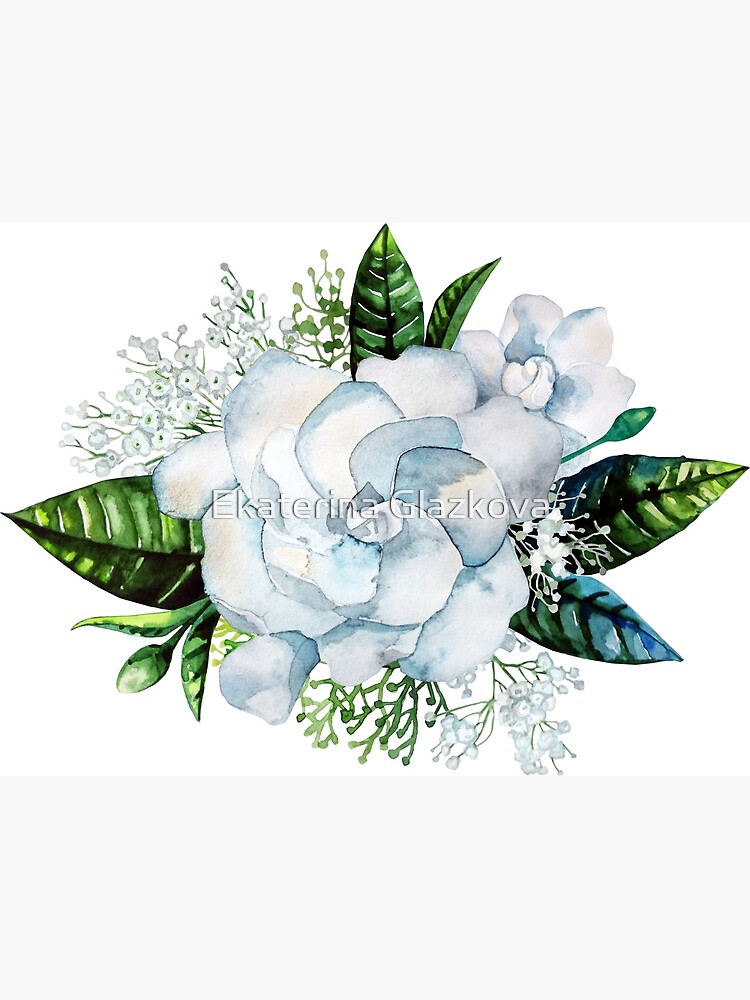This watercolor painting by Ekaterina Glazkova centers on a prominent, large flower with white petals subtly tinted with blue-grey, giving it a soft, serene feel. Surrounding the main flower are lush green leaves, interspersed with sprigs of smaller flowers and buds, which add dimension and texture to the piece. The petals of the central flower are edged with a slight grayish hue, enhancing their delicate appearance. The background remains a pristine white, allowing the detailed botanical elements to stand out vividly. The entire composition maintains a realistic yet distinctly watercolor aesthetic, avoiding hyper-realism. The painting includes a visible watermark of the artist's name, confirming its authenticity. The scene is harmonious, with small blossoms and foliage arranged thoughtfully around the central bloom, creating a balanced and intricate floral bouquet.